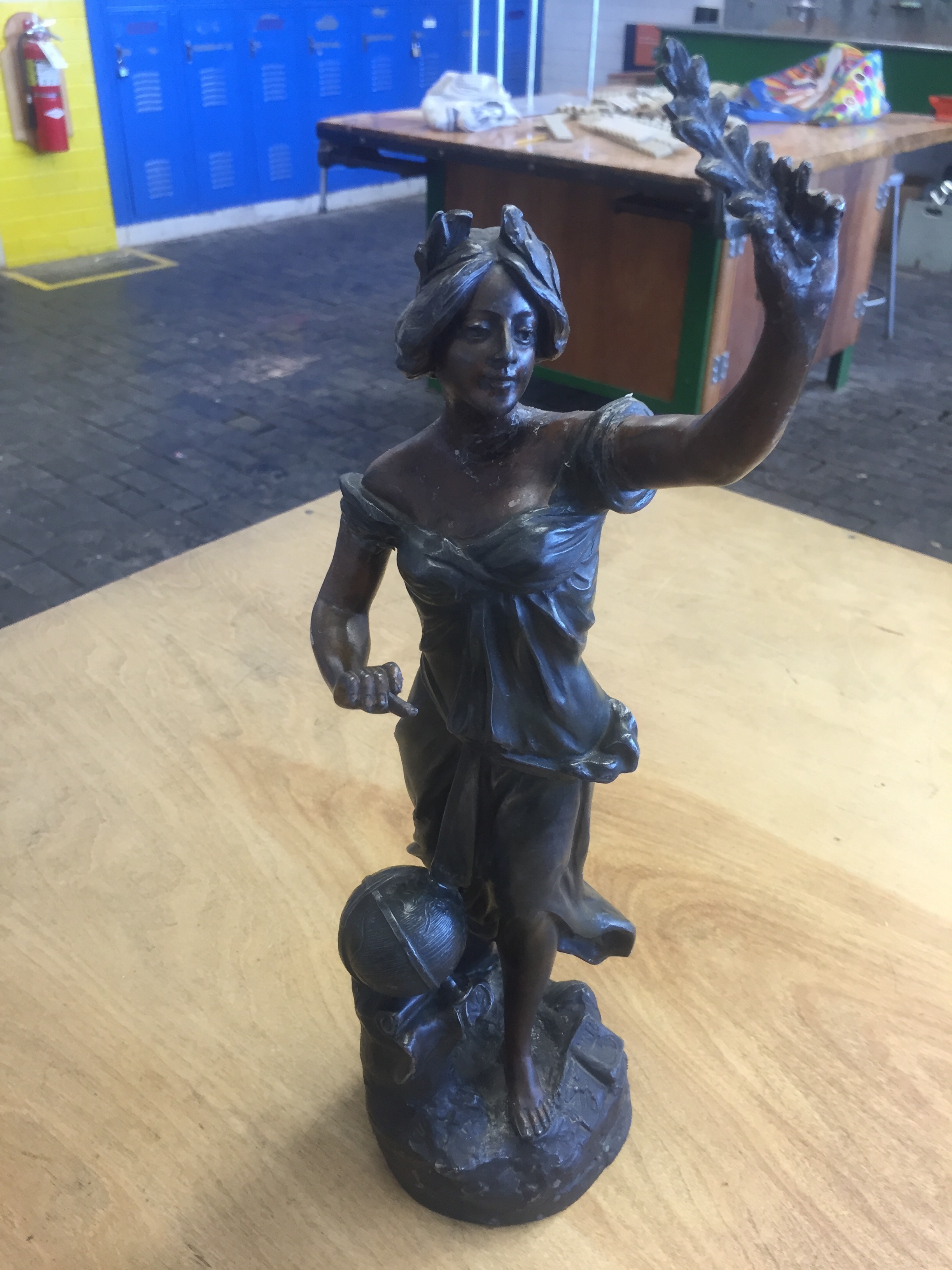This image showcases a close-up photograph of a dark bronze or black-colored statue of a young woman. The statue, finely detailed and appearing to be made of a copper-like material, depicts the woman barefooted and standing on uneven rock with a sphere next to it. She wears a short, robe-like dress that accentuates her form and has her hair styled in an elaborate pile on top of her head. The woman's left hand is extended forward, holding up a tall leaf or branch, while her right hand is making a fist with one finger pointing out.

The statue is positioned on a light yellow wooden desk with a stained design. In the background, there's another wooden table across the room, which appears to hold paper and art supplies suggesting a creative setting, possibly an art class in a school. The room features a stone tile floor and a yellow wall to the left, adorned with a fire extinguisher. To the right of the yellow wall, there is a set of blue lockers, adding to the impression of an educational environment.